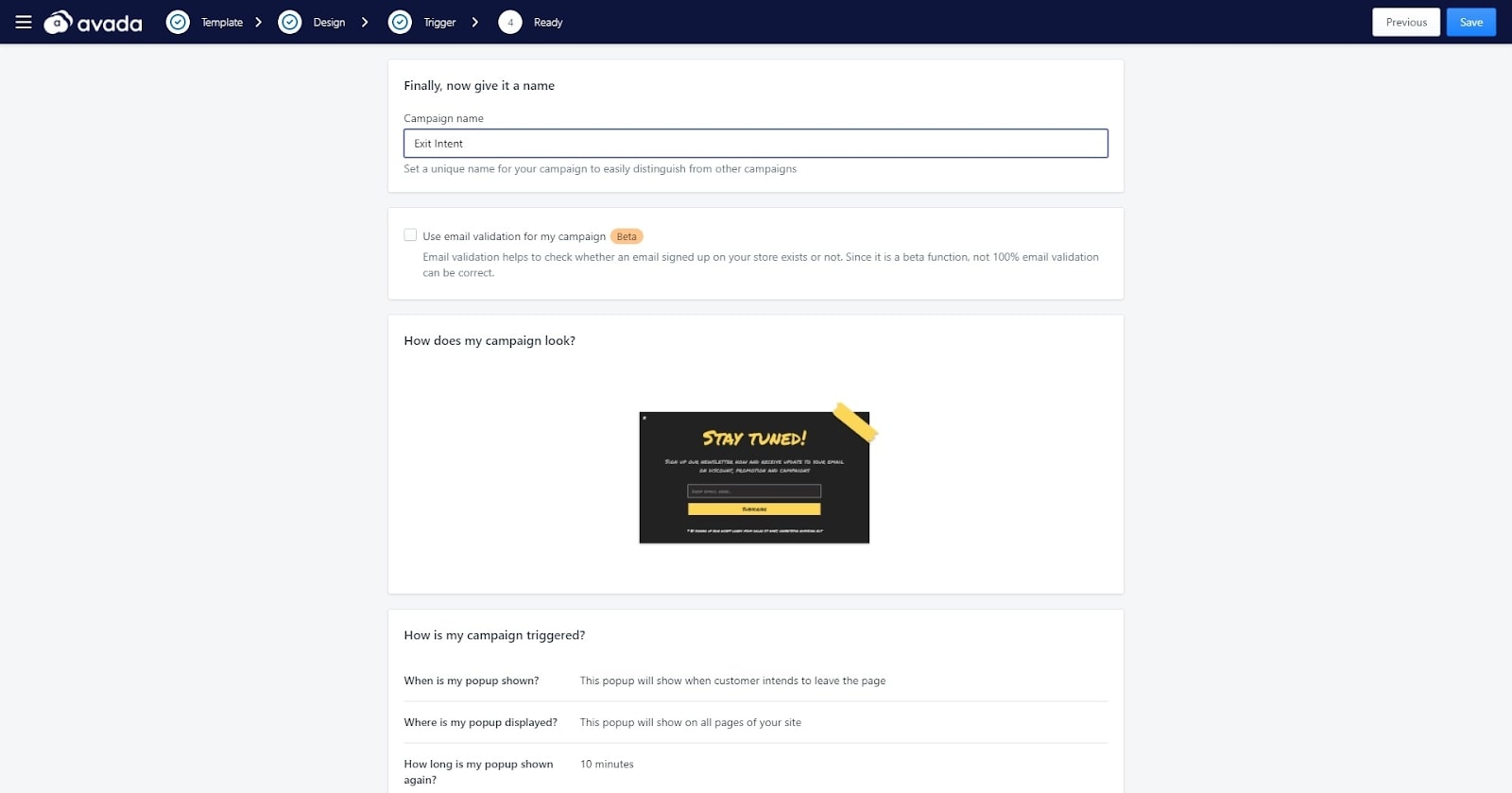This image is a screenshot of a website interface. At the top, there is a black banner featuring white text. In the upper left corner, there is a menu icon followed by a logo resembling a white cloud. Next to the logo, the company name, "Avada," is prominently displayed in bold white text. The navigation menu to the right includes items labeled "Template," "Design," "Trigger," and "Ready," each with a pull-down arrow for further options. 

In the upper right corner, there are two action buttons: a "Previous" button and a "Save" button, with the latter highlighted in blue. Below this banner, a white box contains dark grey text that prompts, "Finally, now give it a name." Within this box, there is an input field for entering the campaign name. Under this input field, there is another labeled box with the text, "How does my campaign look?" in grey.

Further down, a black square displays the message, "Stay tuned," in yellow text. Below this square, another white box asks, "How is my campaign triggered? When is my popup shown?" To the right of this question, it explains, "This popup will show when the customer intends to leave the page."